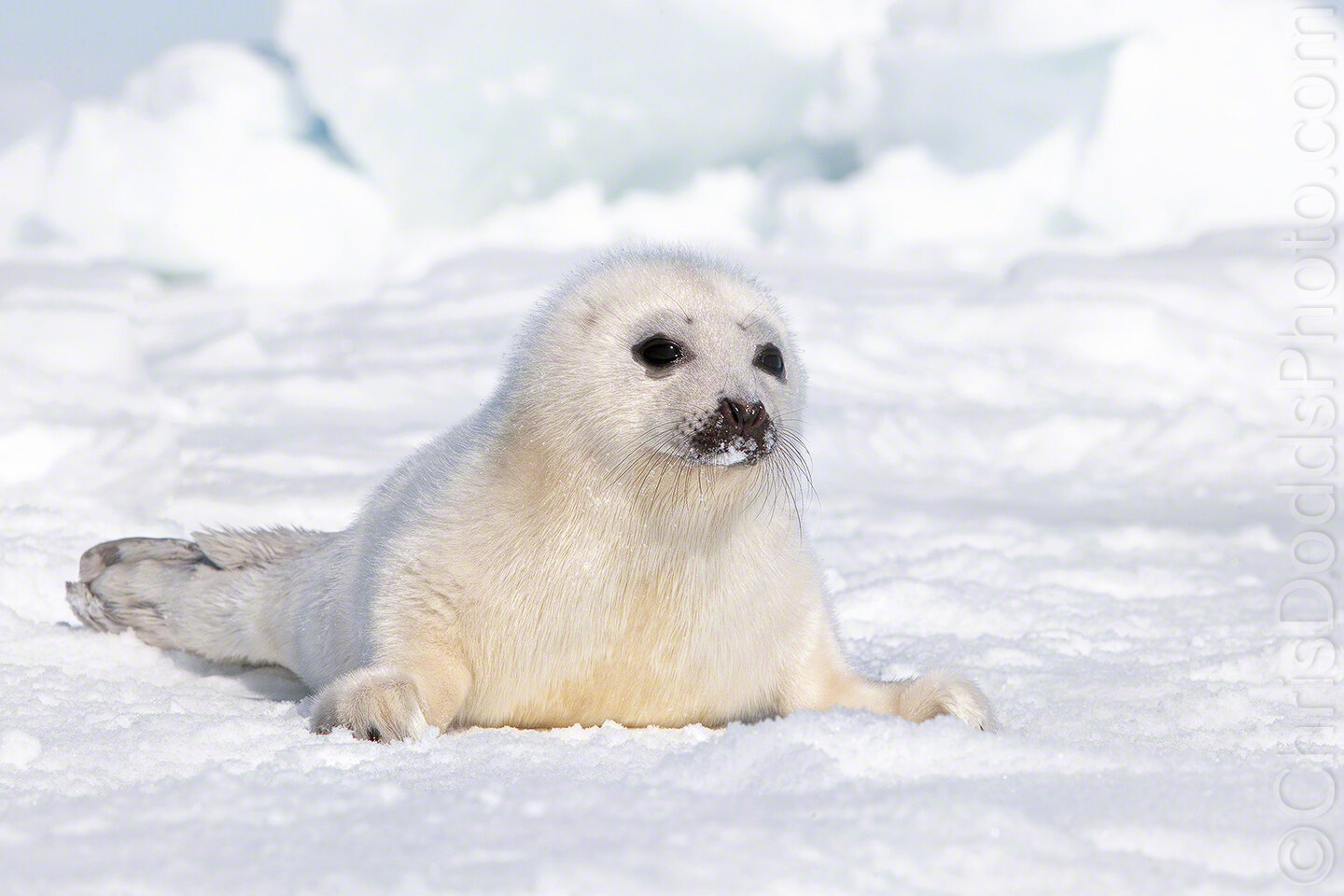In this detailed depiction, the image captures a young white baby seal nestled on a blanket of snow, its serene surroundings depicted in a photographic style. The seal has a cream-colored chest, white head, and features striking black beady eyes with gray whiskers flanking its black snout. A touch of snow dusts its mouth. The front paws are splayed naturally to the sides, and although partially obscured by snow, a dark claw is discernible on the right paw. The background showcases vast expanses and mounds of pristine snow, stretching into the distance. The seal, lying calmly, projects a slightly melancholic expression, perhaps a natural trait of its features. Additionally, there's a subtle watermark on the image's side, possibly reading "CordisDodds.com" in grey, adding to the authenticity of this serene winter scene.